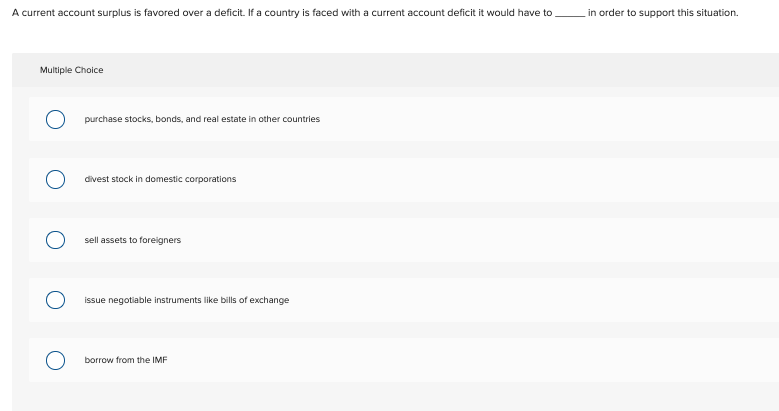Screenshot of a Survey Website: 

The image displays a survey website with an off-white or grayish background. 

At the top of the page, the survey question is prominently featured: "A current account surplus is favored over a deficit. If a country is faced with a current account deficit, it would have to ______ in order to support this situation." 

Below the question, there is a multiple-choice section with various answer options provided to complete the sentence. Each option has a clickable circle outlined in blue and filled with white on the left side, which indicates the area users need to click to select their response. 

The multiple-choice options are as follows:
1. Purchase stocks, bonds, and real estate in other countries.
2. Divest stock in domestic corporations.
3. Sell assets to foreigners.
4. Issue negotiable instruments like bills of exchange.
5. Borrow from the IMF.

All text is presented in a standard black font, maintaining a simple and clear layout. The design and structure of the survey website are quite straightforward, ensuring ease of use for respondents.